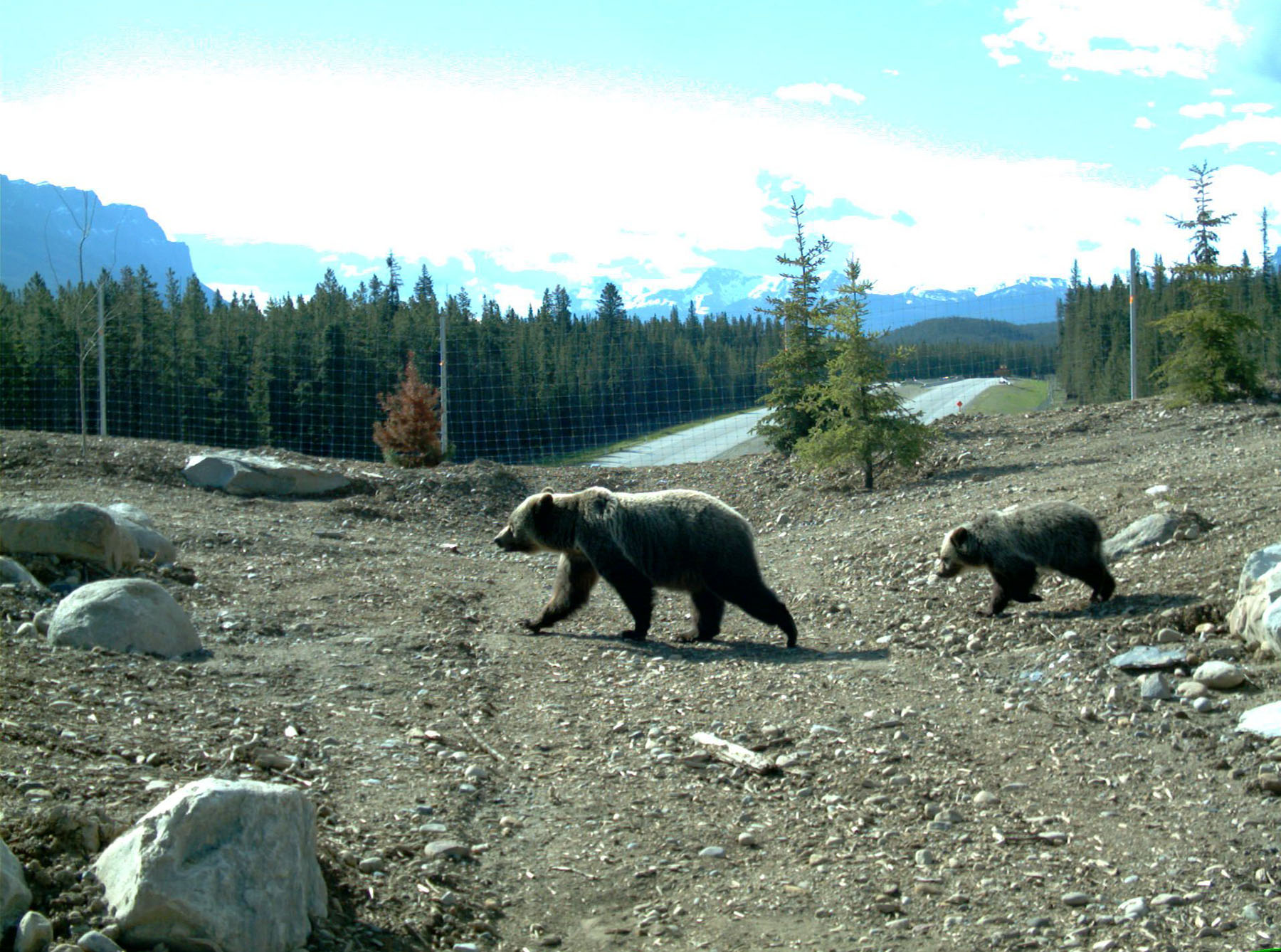The color photograph captures a vivid scene of a grizzly bear and her cub walking across rocky ground. The mother bear, with her left profile prominently displayed, strolls toward the left side of the image, closely followed by her cub just a couple of feet behind. The terrain beneath them is rugged with an abundance of small rocks and a few larger ones jutting out. Their backdrop includes several tall spruce or fir trees, beyond which lies a windowpane mesh metal fence, suggesting a possible enclosure. Farther in the distance, the landscape features rolling hills, a road, and a dense expanse of spruce forest with majestic mountains rising in the background. The sky above is an overexposed aqua blue, filled with indistinct, bright white clouds that blend into one another. This picturesque scene, likely set in Alaska, highlights the natural beauty and simplicity of the wilderness, with the bears as the focal point amidst the varied textures and elements of their environment.